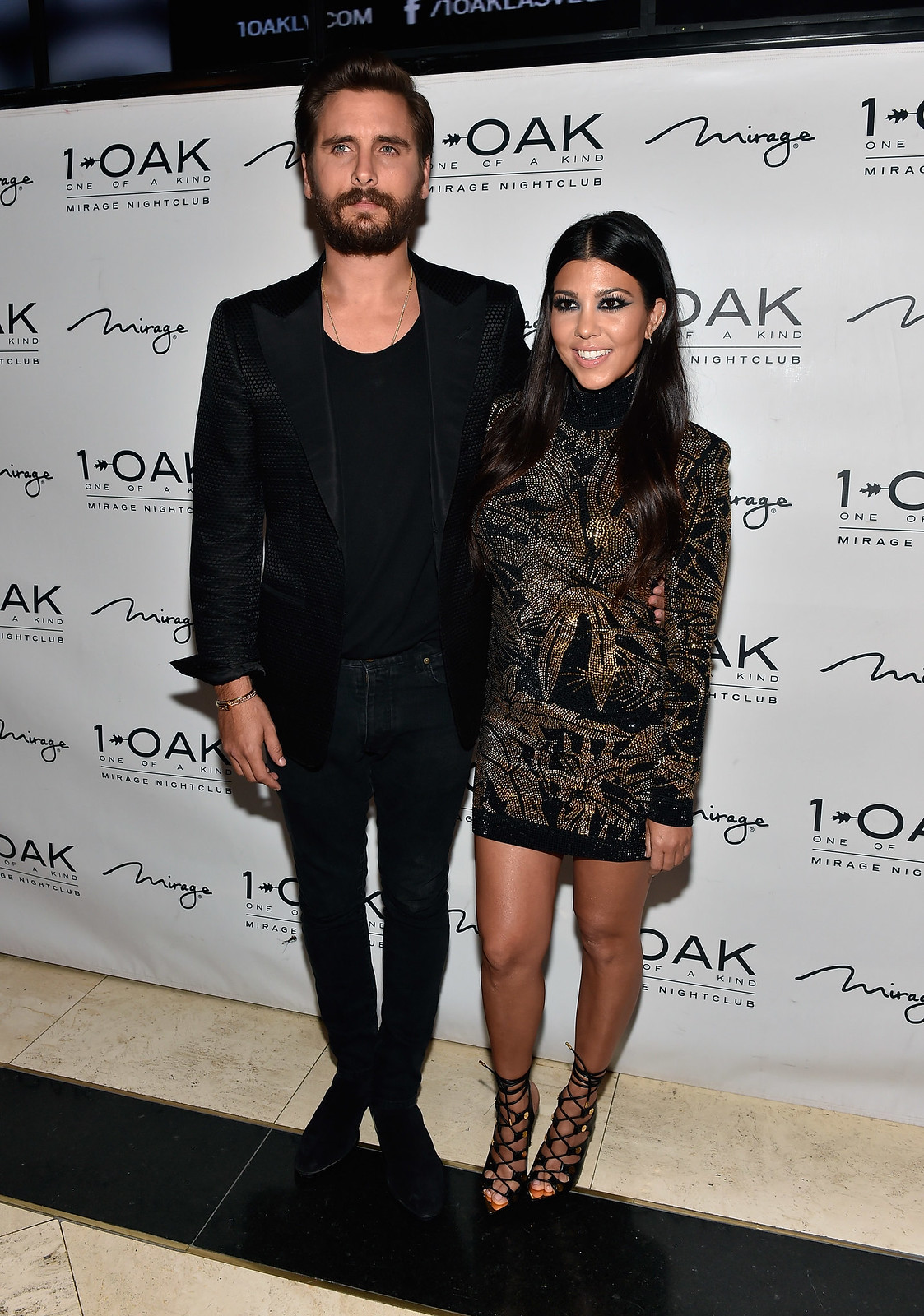In the image, we see Scott Disick and Kourtney Kardashian posing at a red-carpet-style event. Both are standing in front of a white sign with logos saying "One Oak, One of a Kind, Mirage Nightclub" repeated across the background. Scott Disick, who is on the left, is a tall, very thin Caucasian man wearing an all-black outfit consisting of a black blazer, a black t-shirt, black jeans, and black shoes. He accessorizes with a gold chain around his neck and some jewelry on his wrist, while his feet are intriguingly crossed, right over left.

On the right is Kourtney Kardashian, who exudes elegance in a dark thigh-high dress adorned with a gold pattern throughout. She complements her glamorous look with black high-heeled laced shoes. Kourtney has long hair that cascades past her shoulders and is smiling warmly at the camera. The setting appears to be an upscale venue, likely a nightclub or event space, emphasized by the tiled floor and sponsors' signage in the background. The duo is very well-dressed, suggesting they are at a significant event, possibly in a major city like Las Vegas or Los Angeles.